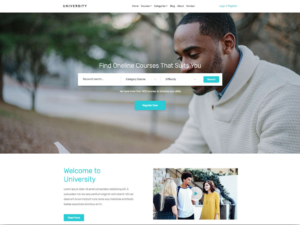This image features a prominently centered, high-resolution photograph of an attractive African American man with neatly lined-up black hair and a well-trimmed short beard. He is wearing a white sweater that features a side button and appears to be gazing down, possibly at a book.

Above the main image, there is some text, and a clickable white bar runs across the top, offering various options. Directly below this bar, there is a large aqua-colored banner which is also clickable, containing the text "Find Online Courses That Suit You."

The setting of the main image appears to be outdoors, with leaves scattered on the ground and trees surrounding the man, suggesting an autumnal environment. Beneath this primary image, there is an additional picture featuring three people. To the left of this secondary image, the text reads "Welcome to the University," adding an inviting touch to the overall composition.